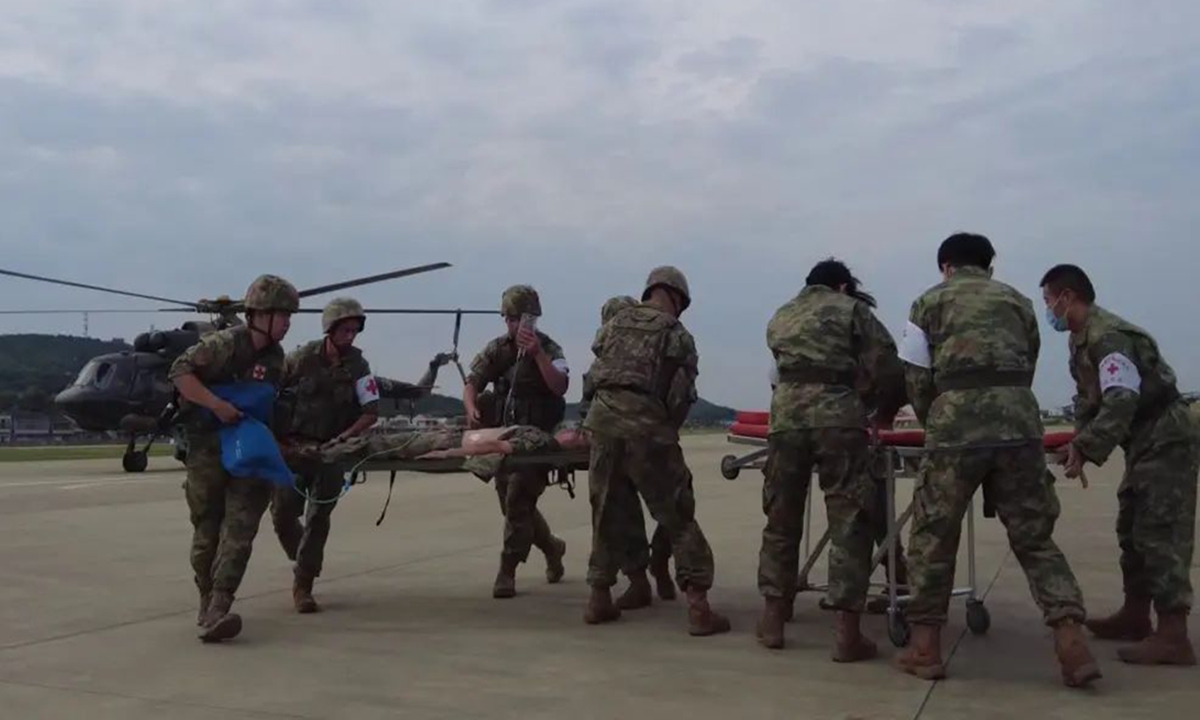This photograph captures a tense medical emergency at what appears to be an Asian army base or flight pad. The scene is populated by at least eight individuals, possibly nine, who are all wearing army camouflage outfits and brown boots. Half of them also have camouflage helmets, while others are without. Focused on their urgent task, these soldiers seem to be medics, distinguished by white armbands with red crosses and some indecipherable writing. 

Central to the image, five soldiers are hurriedly carrying an injured comrade on a makeshift stretcher. One of them is additionally holding a bag of liquids connected to the injured person, indicating medical intervention in progress. To the right, four other soldiers gather around an empty red stretcher, seemingly preparing to assist or transport another casualty. 

In the left middle of this concrete airfield stands a grounded helicopter, possibly the one that transported the injured soldier. The background reveals a sky and some distant hills. All the soldiers appear to be in motion, underscoring the urgency and the live, candid nature of the event taking place.